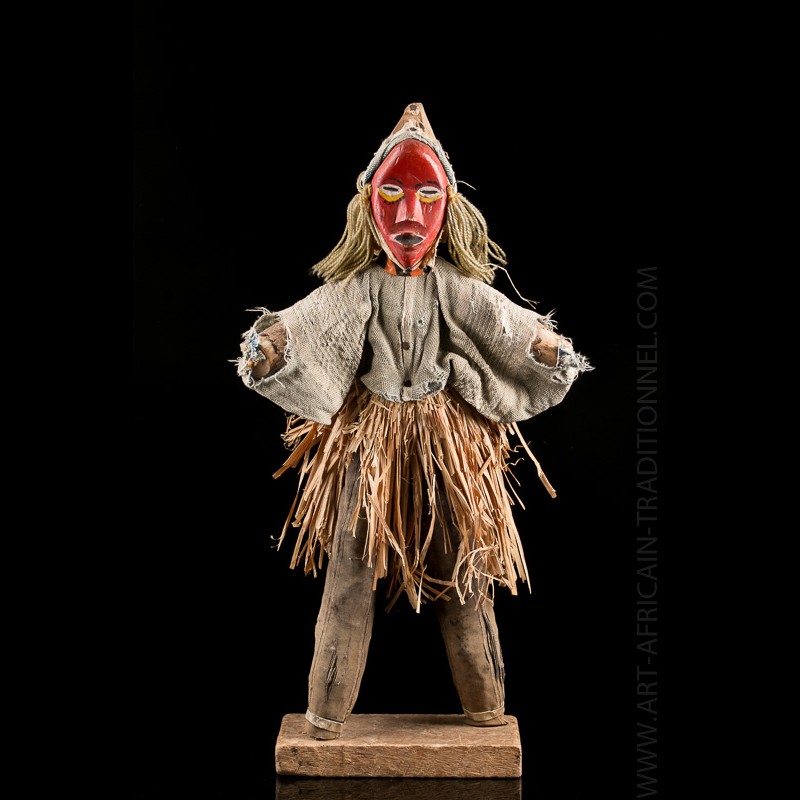The photograph captures an intricately designed doll with a distinct anthropomorphic form placed against a completely black background. The doll's face is a striking red mask featuring black eyebrows, white eyes with black pupils, and brown or yellow curves below the eyes that resemble irises. It has a broad nose and broad black lips on an elongated, oval-shaped face. The doll's hair is represented by threads sprouting from a hat-like triangular top. 

The attire is notably worn and consists of a tattered grey top and ragged brown trousers. Additionally, straws protrude from the upper part of the doll, forming a skirt-like structure. The doll stands firmly on a cubic stone plinth, adding a sense of prominence and stability to the figure. On the right side of the image, the text "www.artafricantraditionelle.com" appears as a vertical watermark, running from the bottom to the top. The entire scene is centered within the frame, emphasizing the unique and detailed craftsmanship of the doll.